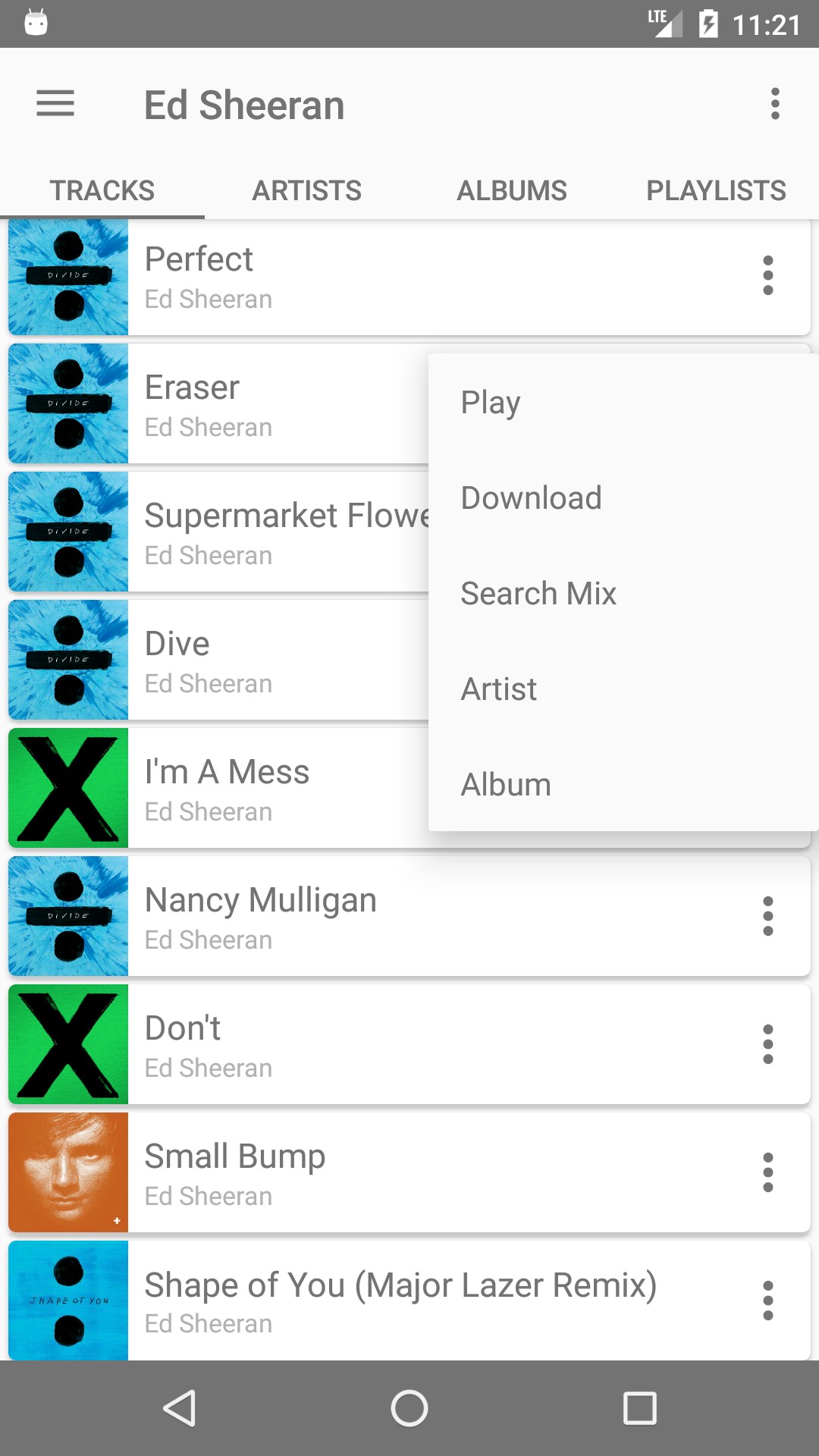Here is a cleaned-up and detailed caption for the image:

---

The image depicts a smartphone screen displaying the YouTube Music app at 11:21 AM. At the top of the screen, the gray phone status bar shows a white "11:21." Below it is the name of the artist Ed Sheeran, followed by four tabs labeled "Tracks," "Albums," "Artists," and "Playlists." The "Tracks" tab is underlined, indicating it's currently selected.

On the left side of the screen, album artwork is visible. Although the speaker does not listen to Ed Sheeran, they describe several tracks featured prominently:

- There is a blue background with two black dots featuring the title "Shape of You (Major Lazer Remix)" in gray text.
- A smaller image above this shows Ed Sheeran’s face with his name below.
- Another track titled "Don't" has a black 'X' on a green background with Ed Sheeran's name.
- The screen shows "Nancy Mulligan" with a divide symbol across the album artwork and Ed Sheeran's name below.
- "Dive" by Ed Sheeran appears next with a similar divide symbol.
- A song titled "Supermarket Flowers," partially obscured, is cut off by another tab.
- Above that is "Eraser," again with the divide-themed background.

The top listed song is "Perfect." The active tab is white with black text reading "Play Donald's Search Mix Artist Album."

---

This caption aims to provide a detailed and structured description of the content displayed on the YouTube Music app on the smartphone screen, focusing on the layout and specific elements visible.